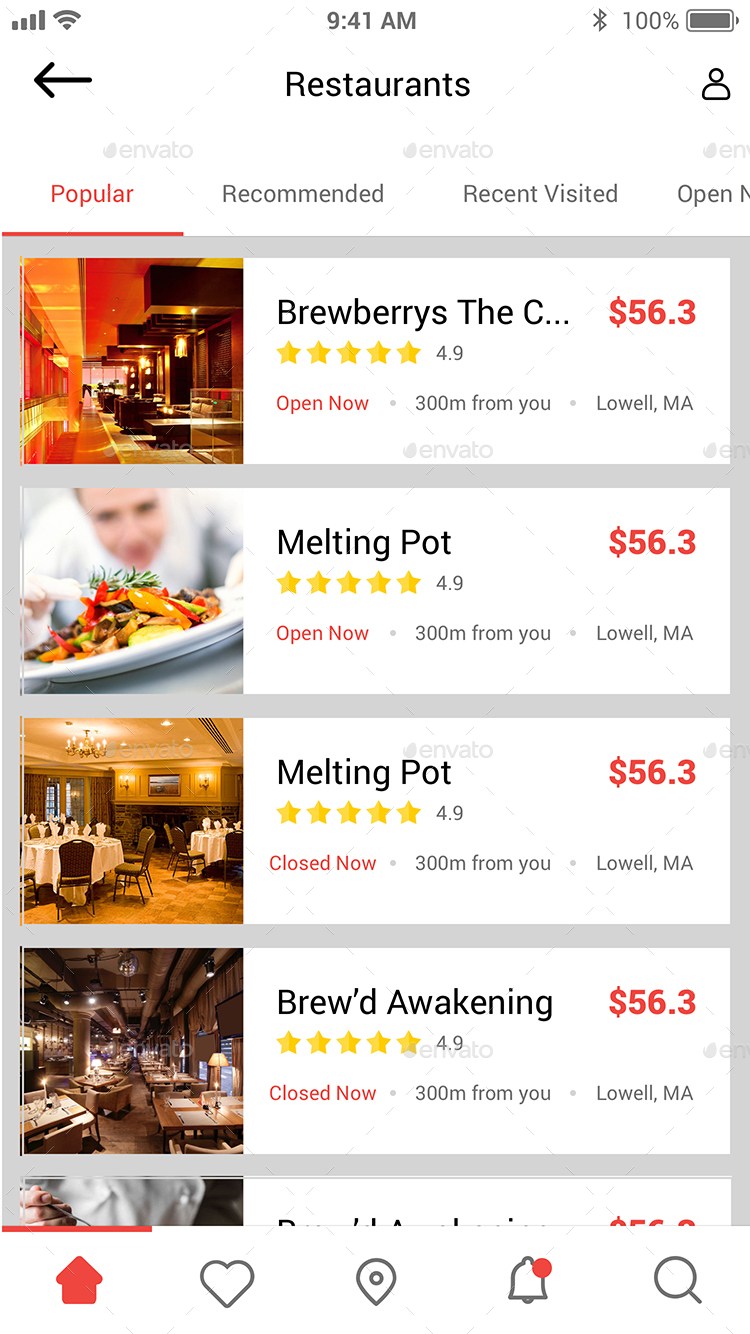The image is a screenshot featuring a smartphone interface set against a white background.

- Top section: On the upper left, icons for cellular reception and Wi-Fi are displayed in black. In the center, it shows the time: 9:41 AM. On the upper right, the battery is fully charged at 100% with Bluetooth enabled.
- Just below this top section, bold black text reads "Restaurants."
- Beneath the main heading, there is a navigation menu with tabs labeled "Popular," "Recommended," "Recent," "Visited," and "Open." The "Popular" tab is highlighted in red.

The main display consists of a list of restaurants showing an image and ratings for each:

1. **Brewberries**
   - Rating: 4.9 stars (yellow stars)
   - Status: "Open now" in red text
   - Image: A sleek, modern, dark-themed restaurant

2. **Melting Pot**
   - Rating: 4.9 stars
   - Status: "Open now"
   - Location: Lowell, Massachusetts
   - Image: A chef holding a beautifully presented plate of food

3. **Melting Pot** (appears again)
   - Rating: 4.9 stars
   - Location: Lowell, Massachusetts
   - Image: Another angle of the restaurant, showing tables and chairs

4. **Brewed Awakening**
   - Rating: 4.9 stars

Each restaurant entry features high-quality images that give a distinct feel of their ambiance or service, catering to the user's interest in dining options.